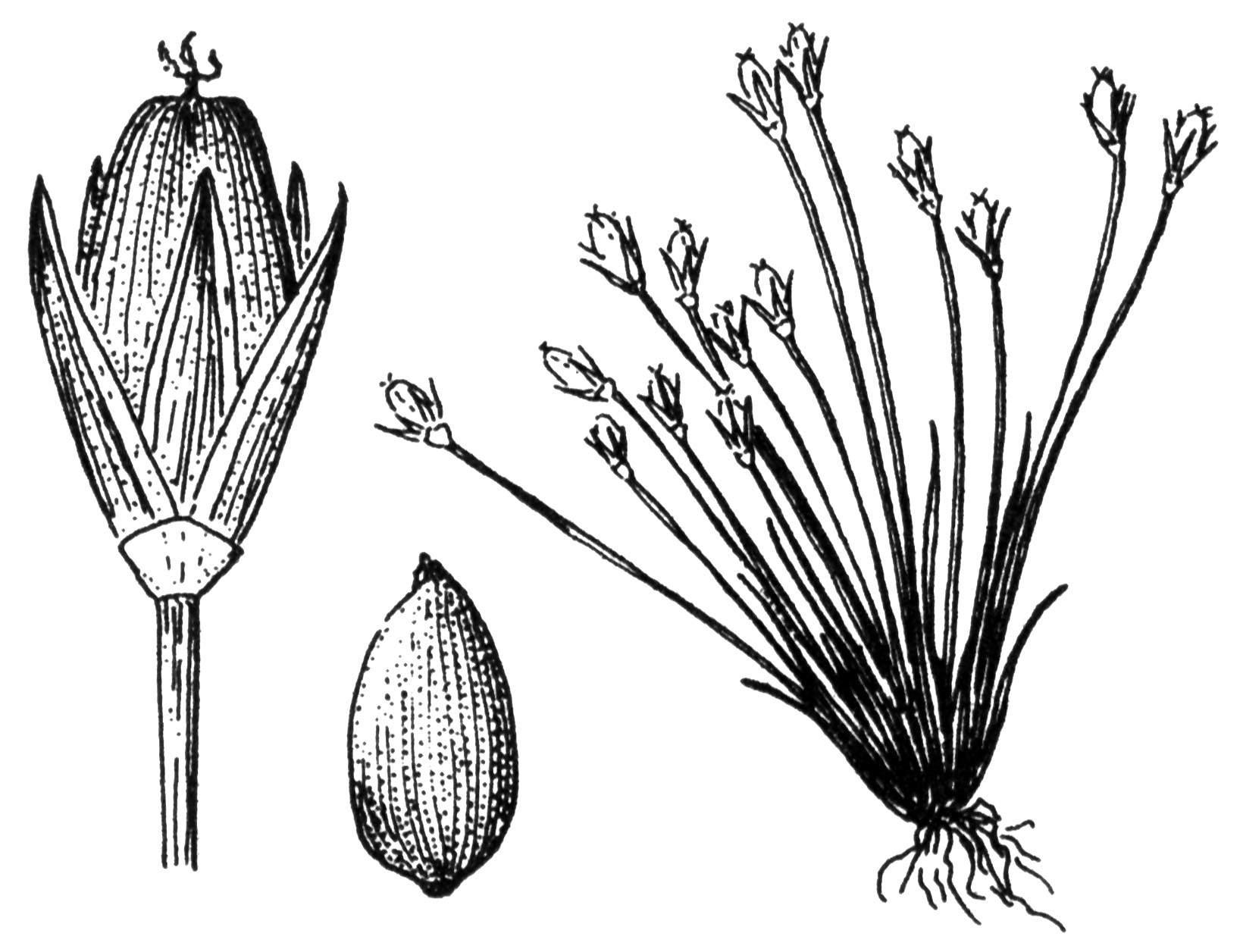This black and white ink illustration is a detailed botanical sketch that features three stages of flower development. On the left, there is a close-up depiction of a flower bulb starting to open. The bulb sits atop a single stem, with five slightly fanned petals and a flat-topped center that has three small hairs growing out of it. The middle sketch portrays the flower bulb in a fully closed state, resembling the texture and shape of an almond or corn cob. On the right side, the illustration shows the entire flower in full bloom from a distance, complete with long stems holding multiple oval-shaped bulbs, each topped with tiny hairs. The sketch also includes the flower's roots extending into the ground, showcasing the organism's full anatomy and growth stages.